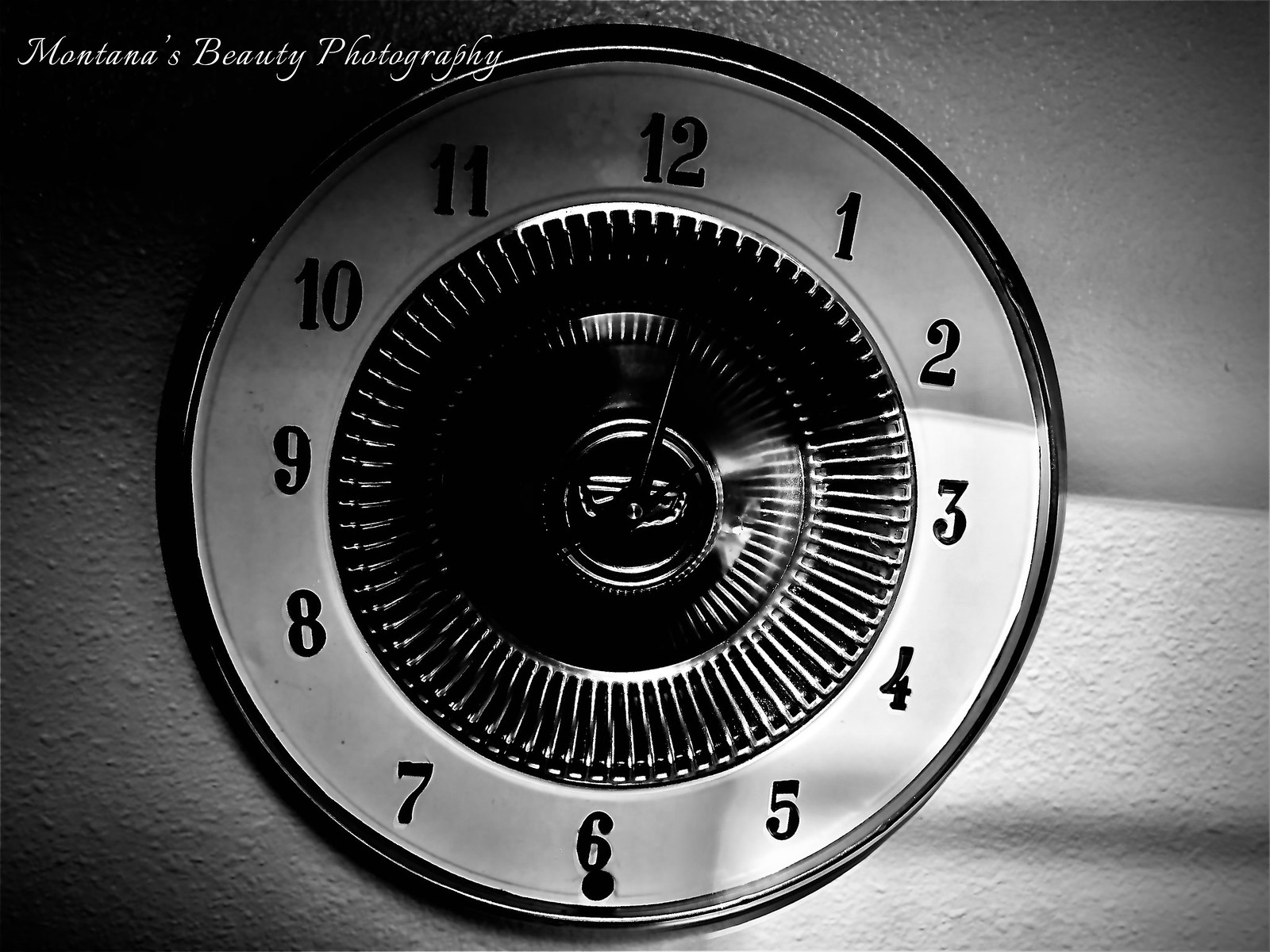The image features a black and silver wall clock, captured with a distinct metallic hue. The clock is framed within a black border and set against a white, stucco-like wall, with light filtering in from the right side. Positioned in the top left corner is a caption in white text, indicating "Montana's Beauty Photography," suggesting the company that produced the image. The clock face displays all twelve numbers, 1 through 12, arranged in a traditional circular fashion. At the center, a radial dial mimicking the texture of a metal grate is present, adding to its vintage aesthetic. The clock hands, though initially hard to distinguish, are visible: one points slightly past the 12, another between the 7 and 8, indicating a time around 7:02, with a ticking second hand situated between the 1 and 2. The overall look is dark and somewhat reflective, evoking the appearance of a stylish, old-fashioned analog device.